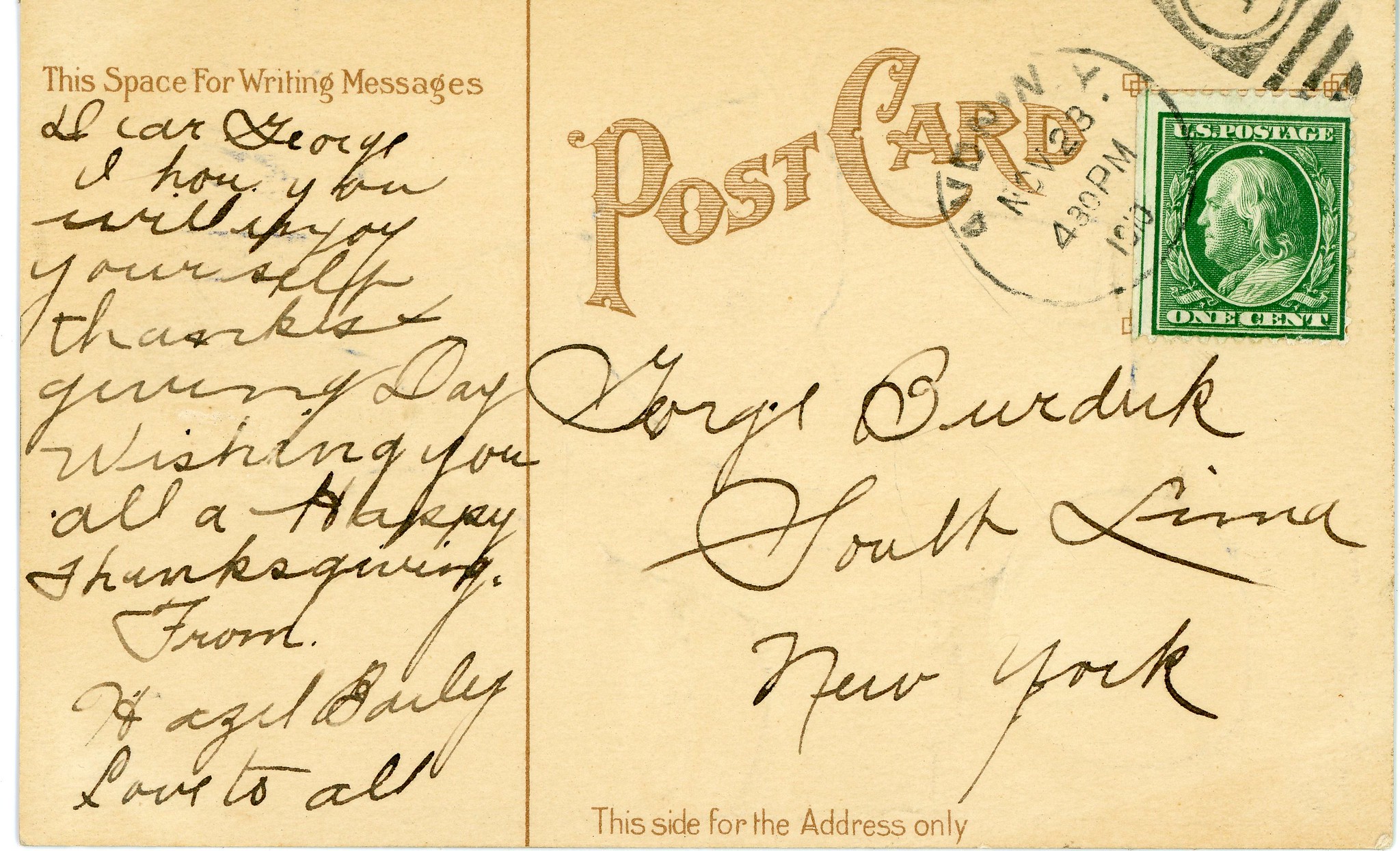This image depicts the back of an aged and yellowed vintage postcard with a cream background, accented by a patina of age. The postcard is divided into two sections. On the left-hand side, there's yellowy-gold text that reads, "This space for writing messages," accompanied by a handwritten cursive note in black ink. The note appears to be addressed to George Burdick and reads, in part, "Dear George, I love you. Wishing you all a happy Thanksgiving from Hazel Bailey. Love to all." The writing is somewhat messy and difficult to decipher in some areas. On the right-hand side, ornate text in the same light golden hue spells out "Postcard." Beneath this is the address "George Burdick, South Lima, New York," written in handwriting, and a reminder at the bottom that reads, "This side for the address only." In the upper right corner, there is a green, one-cent U.S. postage stamp featuring Benjamin Franklin, alongside a black post-date stamp marked November 23rd at 4:30 p.m.